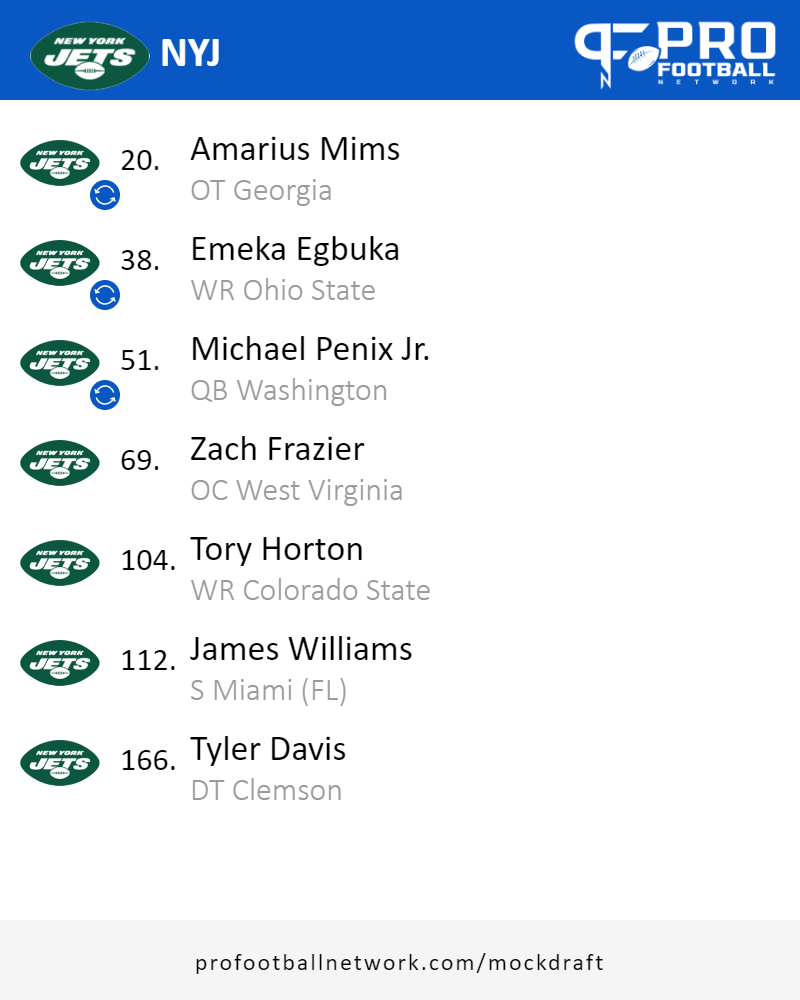The image features a white background dominated by a prominent blue box at the top. Within this box, there is a green football icon emblazoned with the words "New York Jets" written in white. Additionally, the football displays the initials "NYJ" and the acronym "PF" for Pro Football Network. A small football graphic and the word "Network," both in white, are situated towards the bottom.

Below, the graphic lists several player names and details, formatted as follows:

1. A circular icon with two curved arrows in blue, followed by the inscription "#20 Amarius Mims, OT, Georgia."
2. An identical blue circle, followed by "#38 Emeka Egbuka, WR, Ohio State."
3. Another blue circle, then "#51 Michael Penix Jr., QB, Washington."

The listings continue without the circular icons:

4. "#69 Zach Frazier, OC, West Virginia."
5. "#104 Torrey Horton, WR, Colorado State."
6. "#112 James Williams, RB, Miami, Florida."
7. "#166 Tyler Davis, DT, Clemson."

Each listing features the green football icon with the Jets insignia. At the very bottom of the image, a blue box displays the URL "profootballnetwork.com/mockdraft" in white text.